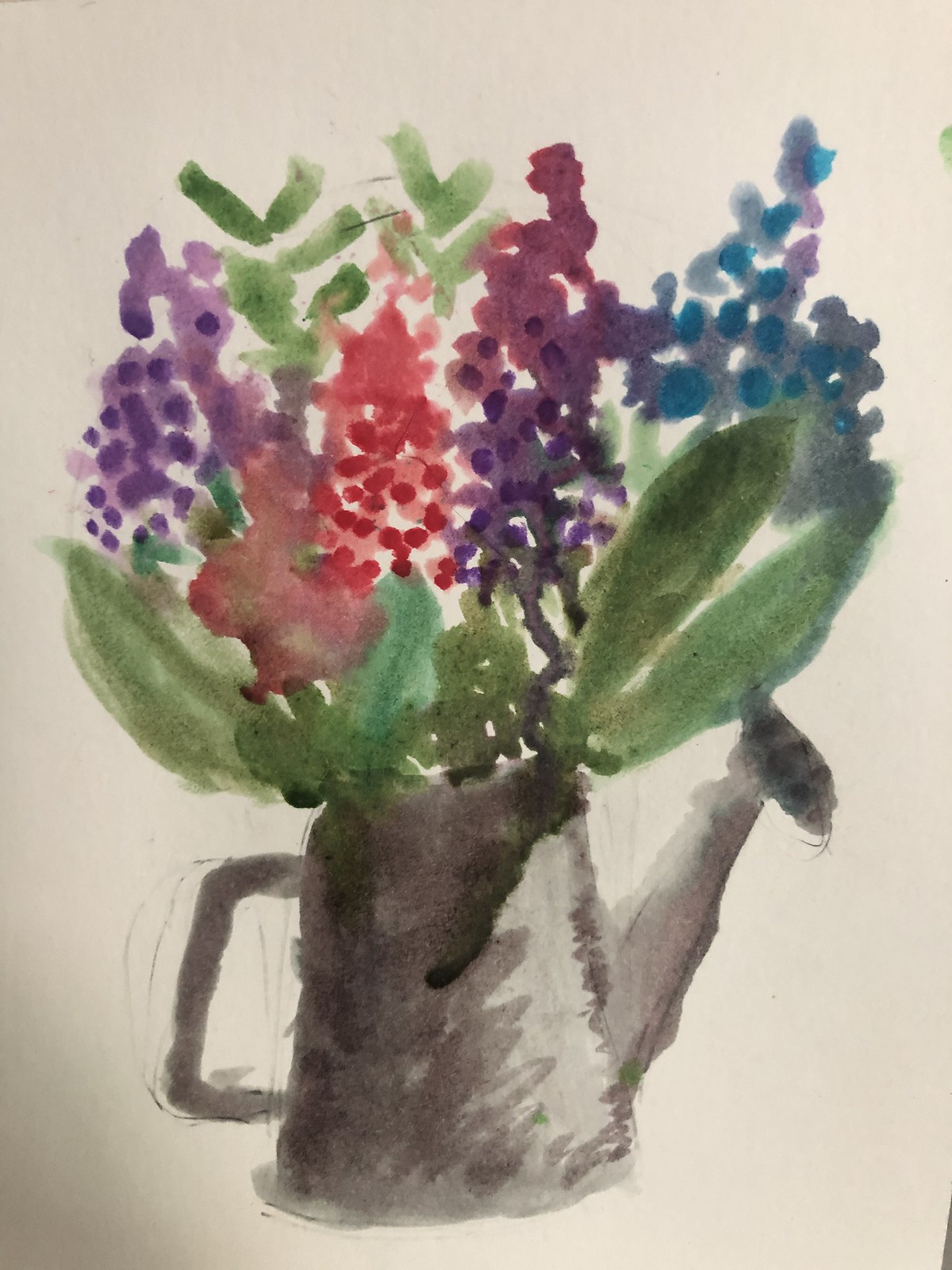This watercolor painting features a side view of a gray, metallic watering can with a bouquet of four flowers artistically arranged inside. The watering can is detailed with a handle and a spout, which is fitted with a circular, perforated nozzle for dispensing water. The bouquet consists of vibrant, hyacinth-like flowers in varying shades: one purple, one red, one deep purple, and one blue, complemented by tulip-like leaves and smaller green foliage. The artist has skillfully used contouring and shadows in shades of gray to give the watering can a three-dimensional, realistic appearance.